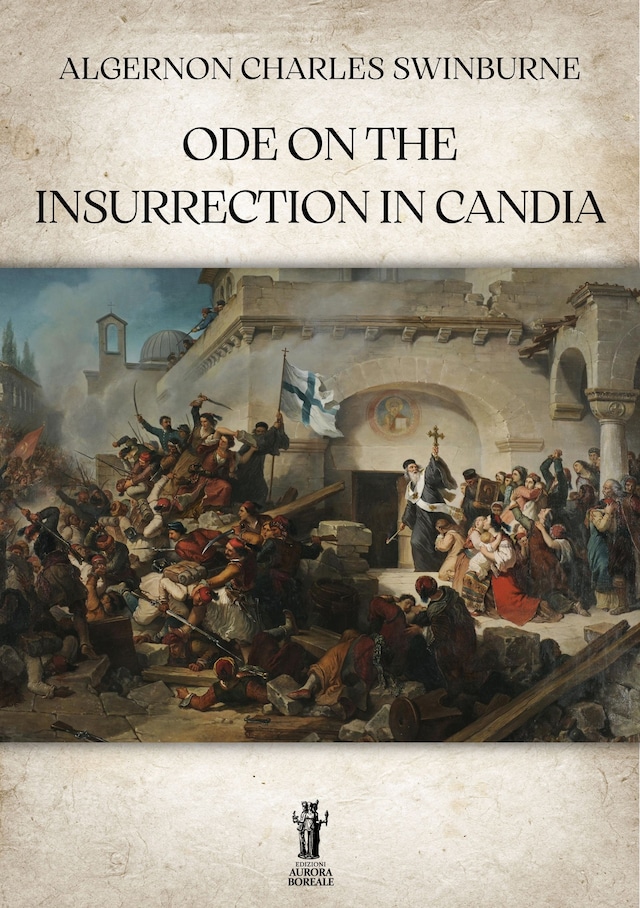This is a book cover featuring a painting-style illustration set outdoors. The book's title, "Ode on the Insurrection in Candia," is prominently displayed beneath the author's name, Algernon Charles Swinburne, both written in capital black letters at the top. The cover art depicts a dramatic historical scene centered around a church. In the foreground, a priest dressed in black robes with a white banner holds a cross aloft, leading a procession of men and women in robes who are praying to him. This group is located in the bottom right corner.

In the middle of the painting, the church with an arch is the focal point. To the left, a man holding a blue and white cross stands alongside another man mounted on a horse and wielding a sword, followed by another sword-wielding man. Below them, additional people, some armed with spears and others lying down, indicate a fierce battle scene. A soldier with a bayonet is seen trying to stab someone amidst the chaos.

The top right-hand corner of the image features another arch, adding to the architectural elements of the setting. The top left corner showcases a blue sky with a tower. At the bottom of the cover, in the center, there is a black and white logo depicting two statues, accompanied by the text "Edizioni Aurora Boreali." The entire cover has an off-white background with light gray splotches, giving it an aged appearance.